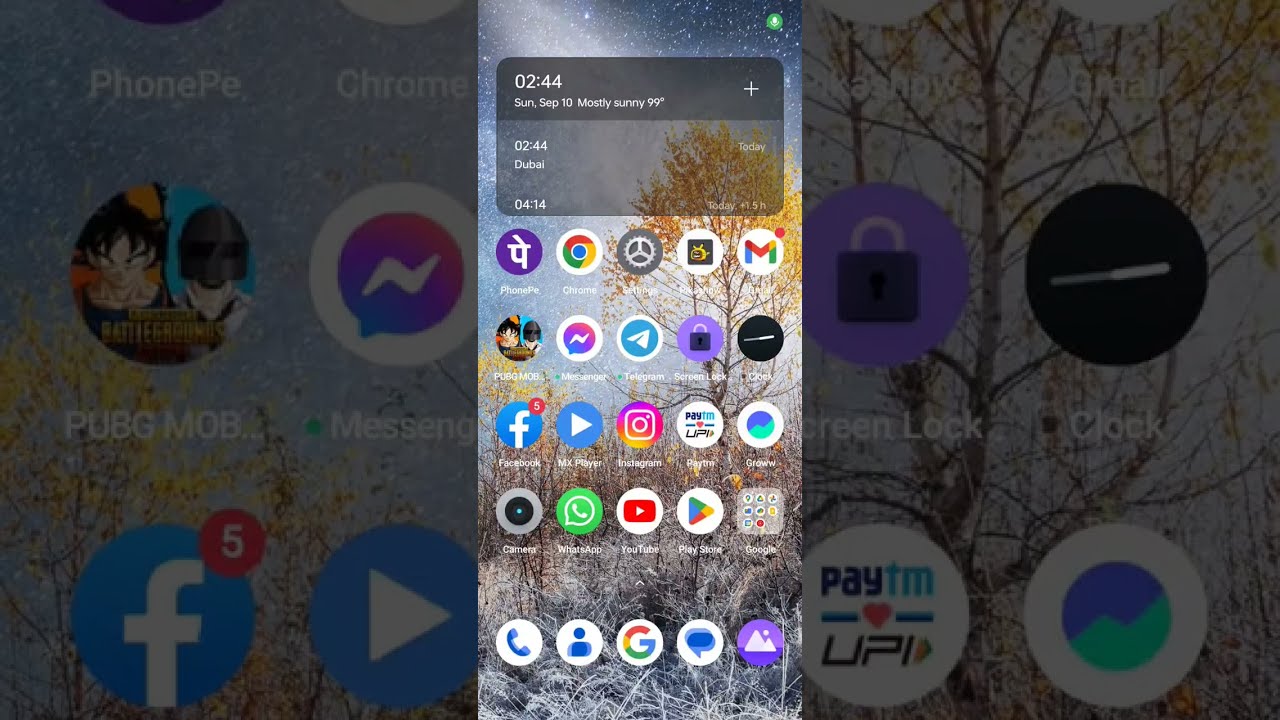The image is divided into three vertical sections: the first and third sections are darkened close-ups of the middle section. The middle section is a detailed screenshot of a mobile phone home screen. At the top of the screen, the device displays the time "2:44 AM," the date "Sunday, September 10th," the weather status "Mostly Sunny," and the temperature "99 degrees," with the location marked as "Dubai." Below this, the screen shows an array of approximately 20-25 app icons, including easily recognizable apps such as PhonePe, Chrome, Settings, Picasso, Gmail, PubG, Messenger, Telegram, ScreenBlock, Cloak, Facebook, MX Player, Instagram, Paytm, Grow, Camera, WhatsApp, YouTube, Play Store, and Google. At the bottom of the screen, there are five icons for calling, contacts, Google search, messaging, and the photo gallery. The wallpaper features a ground area covered with dry grass, a yellow-leaved tree, and a star-filled sky.